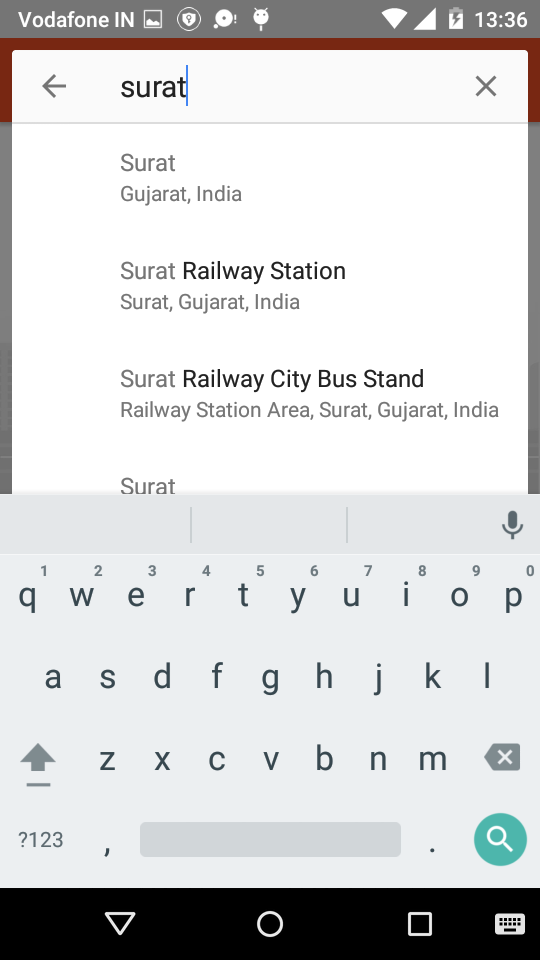This screenshot, captured on a cell phone, displays an active typing session within a search function. Dominating the lower part of the screen, the gray keyboard is visible with a green circle bearing a search icon located at its bottom-right corner and a microphone symbol at the top-right, indicating voice search capability. Just above the keyboard, a pop-up box shows the partially entered term "Sirot," with a blinking cursor positioned to the right of the "T," suggesting ongoing typing.

Directly below this, autofill suggestions list popular searches, including "Sirot Guwarat, India," "Sirot Railway Station in India," and "Sirot Railway City Bus Stand." The remaining suggestions are obscured by the keyboard. At the very top of the screenshot, indicators reveal the phone is using Vodafone service. Additional icons displayed from left to right include a photo gallery, music app, Wi-Fi connection, signal strength, battery level, and the current time.